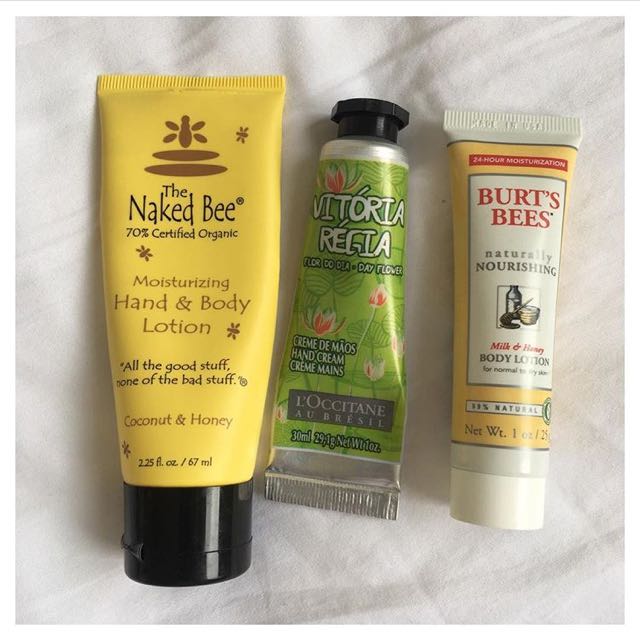The image showcases three distinct hand and body lotions laid out on a white sheet backdrop. On the left, there's a yellow bottle of Naked Bee, featuring a brown bee insignia, with a black cap. It's labeled as 70% certified organic moisturizing hand and body lotion, highlighting ingredients like coconut and honey. In the center, there's a green bottle of Victoria Regia Dayflower Hand Cream, adorned with illustrations of green lily pads and pink flowers; it too has a black cap and a silver base. The bottle on the right is a plastic container from Burt's Bees, distinguished by its yellow and white design, red text, and a white cap. It describes the product as Naturally Nourishing Milk and Honey Body Lotion.